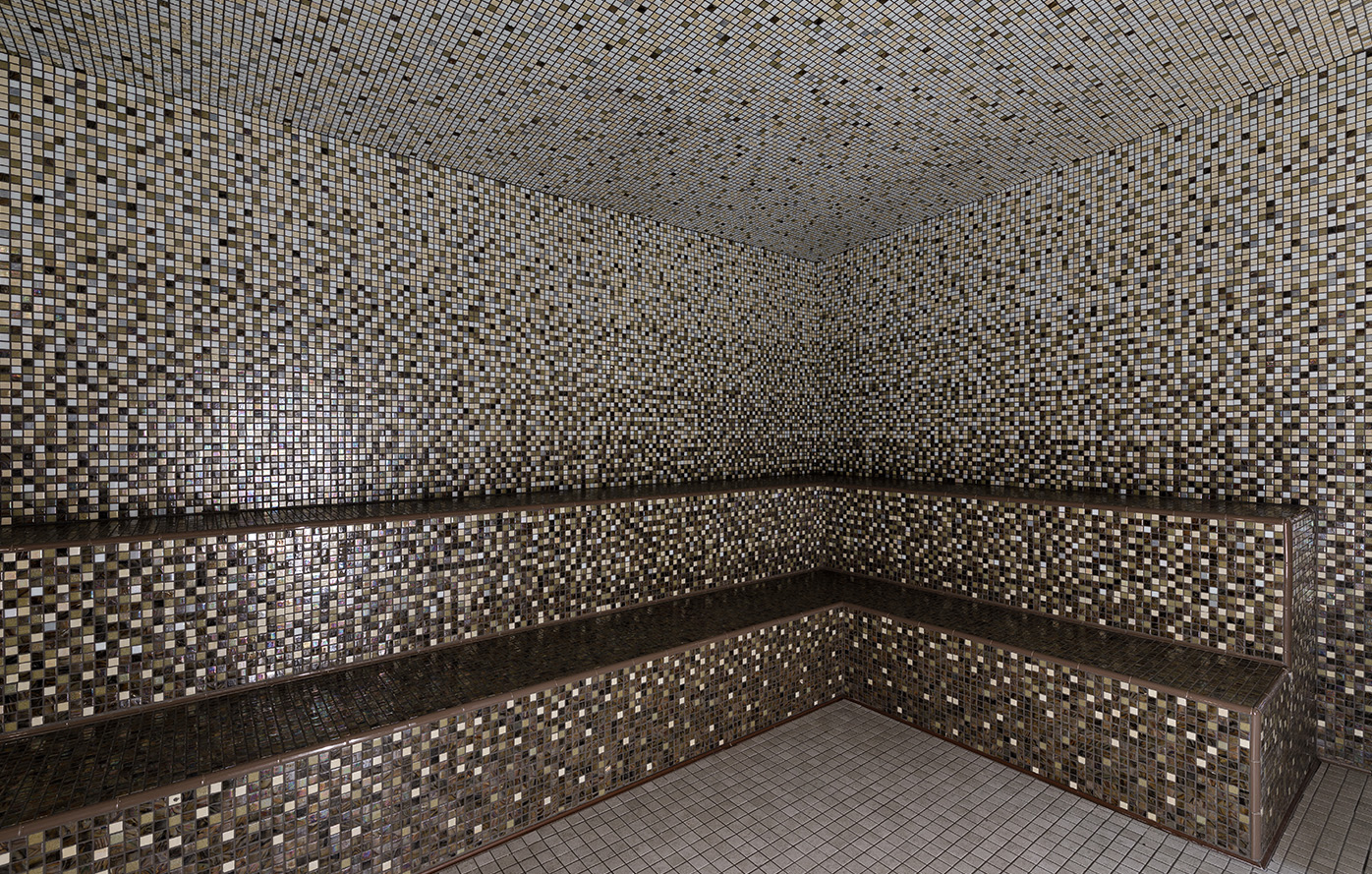The photograph captures the intricate design of an indoor room that appears to be a sauna or steam room, emphasizing the meticulously tiled surfaces that dominate the space. The room is rectangular, with its back corner in view, and features hundreds, possibly thousands, of small tiles in a monochromatic palette of black, white, beige, brown, and gray. These tiles create a striking, almost hypnotic pattern on the walls, ceiling, and floor, gradually transitioning from darker tones near the floor to lighter shades near the ceiling.

The floor is adorned with light gray tiles, while the seating arrangement includes two rows of benches covered in darker tiles. The lower bench, extending from the left and curving into an L-shape towards the center, is decorated with brown and black tiles. Directly above it is a second level, similarly tiled, creating a stepped seating area that allows for sitting or reclining. 

A subtle light source from the right side of the room illuminates the tiles on the left, adding a dynamic element to the mosaic-like pattern. The ceiling features predominantly white tiles with interspersed light brown and black accents, enhancing the room’s unique, cool aesthetic.